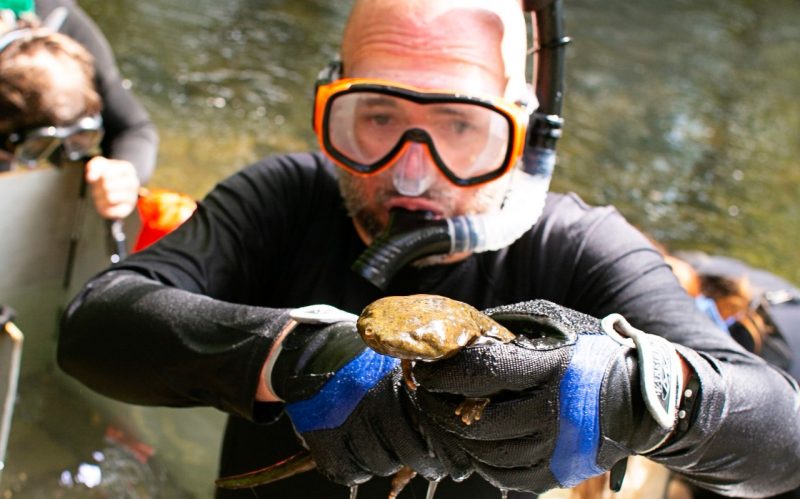In this detailed photograph, a diver is prominently featured, visible from the waist up against the backdrop of a large body of water, potentially a river, ocean, or sea. Illuminated by bright daylight, he stands on a boat, evidenced by a partially visible silhouetted figure in the background. The man is clad in a soaking wet, long-sleeved black wetsuit and thick black gloves with gray Velcro adjustable wrist straps. His headgear includes a black and see-through snorkel secured in his mouth and a pair of swim goggles with a see-through nosepiece and clear lenses in an orange and black frame. In his gloved hand, he proudly displays a flat, green-looking amphibian characterized by its large, bulbous head and tiny fingers that hang in round balls.